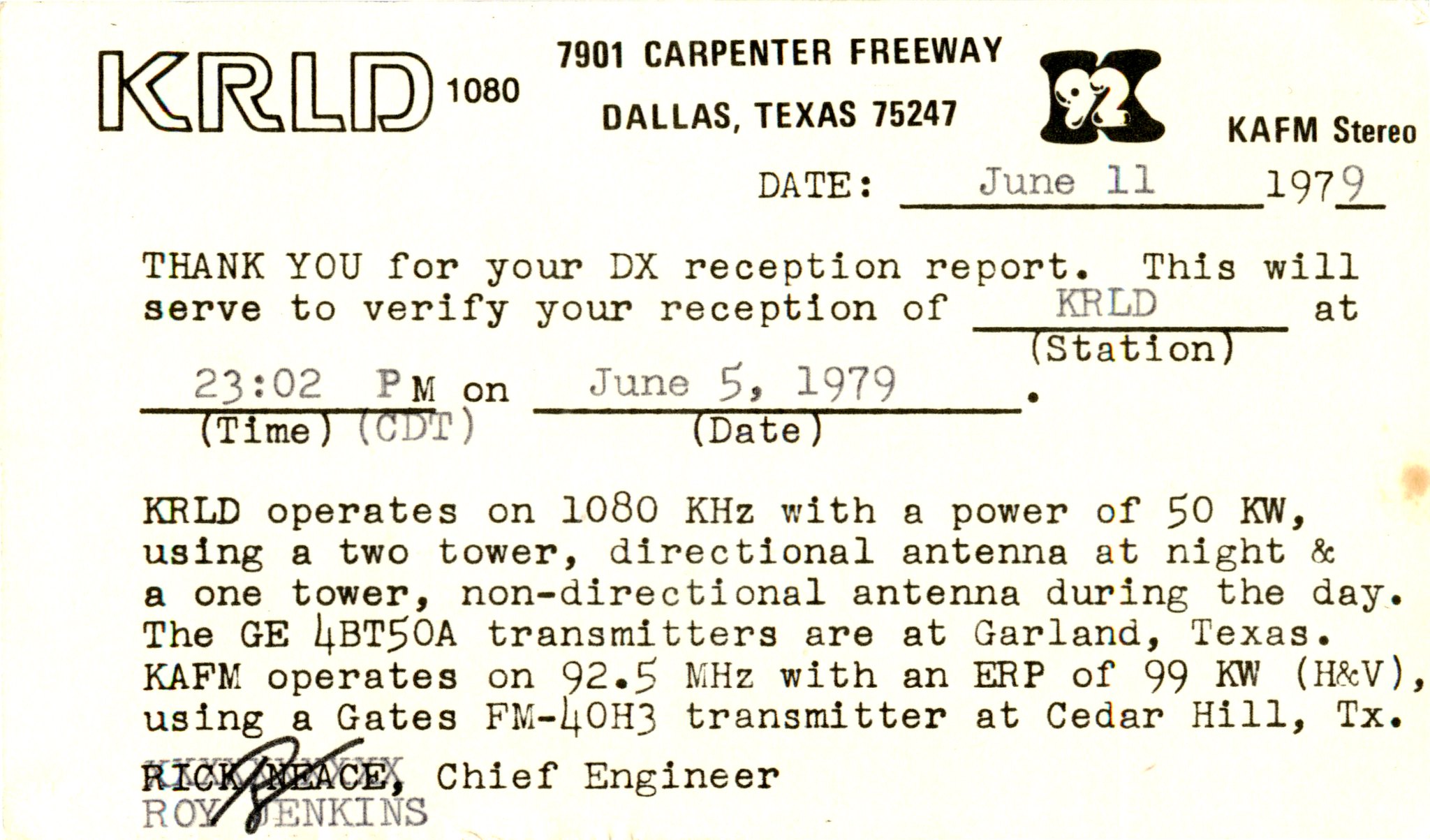The image depicts an official, dated document from June 11, 1979, featuring KRLD in block writing at the top left corner, followed by 1080. In the middle top, there's an address: 7901 Carpenter Freeway, Dallas, Texas, 75247. The document acknowledges a reception report with the statement: "Thank you for your DX reception report. This will serve to verify your reception of KRLD station at 23:02 PM on June 5, 1979.” It details that KRLD operates on 1080 KHz with a power of 50 kW, utilizing a two-tower directional antenna at night and a one-tower non-directional antenna during the day. The GE 4BT 508 transmitters are located in Garland, Texas. Additionally, the document states that KAFM operates on 92.5 MHz with an ERP of 99 kW using a Gates FM-40H3 transmitter at Cedar Hill, Texas. The document is signed by the chief engineer, Boyd Jenkins.